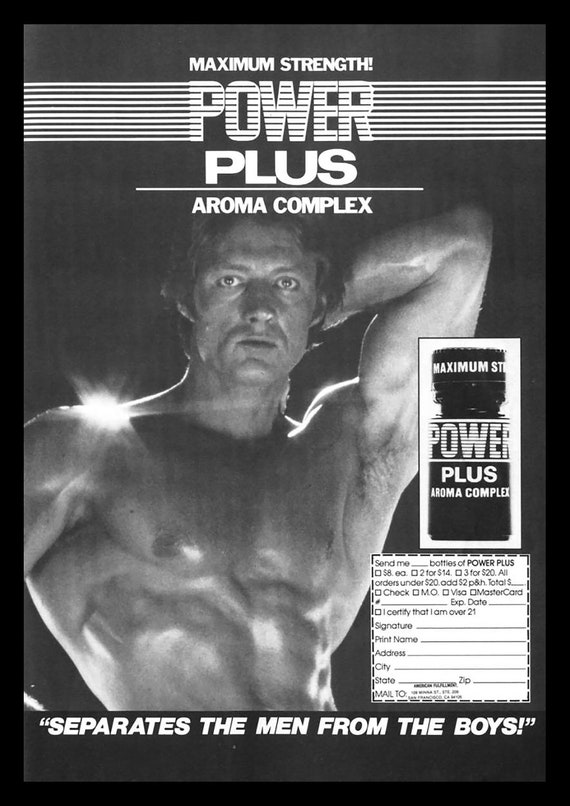An old black-and-white advertisement for Maximum Strength Power Plus Aroma Complex features a highly muscular male bodybuilder with short, curly brown hair and an intense expression. The man poses with his left hand behind his head, showcasing his impressive muscles and abs. The headline at the top reads "Maximum Strength Power Plus Aroma Complex," with the word "power" emphasized by lines radiating from it, suggesting action. To the right of the bodybuilder is an inset image of a small black bottle labeled with the same product name. Below this, there's a coupon section featuring a fill-in form for ordering the deodorant at various prices—one bottle for $18, two for $14 each, or three for $20 total—accepting cash, check, or money order. The bottom of the advertisement contains the slogan "Separates the men from the boys," underscoring the product's appeal to masculinity and strength.